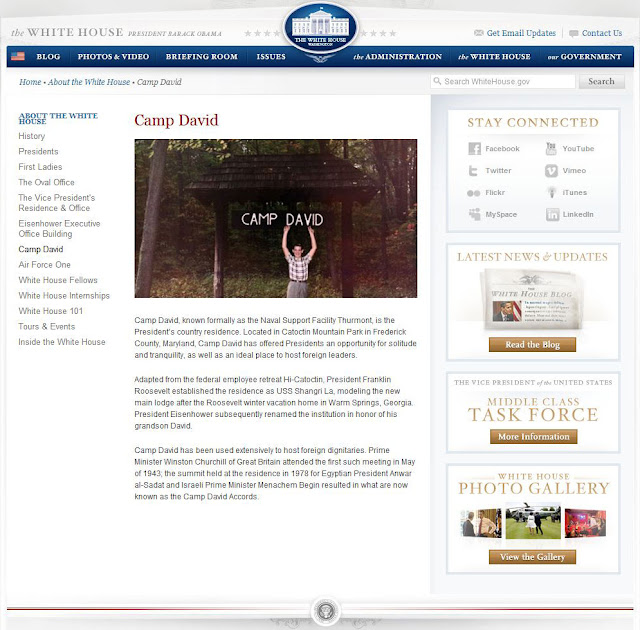The image features a webpage displayed on a computer screen that highlights information about Camp David, a presidential retreat. The webpage belongs to the White House during President Barack Obama's administration. At the top of the page, the White House seal is prominently displayed— a blue oval featuring an image of the White House. The top right corner offers options to 'Get Email Updates' and 'Contact Us.'

A blue navigation bar runs horizontally across the page, displaying an American flag on the left and white text navigation options: Blog, Photos & Videos, Briefing Room, Issues, The Administration, The White House, and Our Government. Below this bar, the page transitions to a lighter color scheme.

In the central section of the webpage, there's a headline that reads "Camp David," accompanied by a photograph. The image shows a person standing in a wooded area, holding up a sign that says "Camp David." Beneath the photo, three paragraphs provide detailed information about Camp David.

To the left of this main content area is a white sidebar containing a list of navigational links. These links, from top to bottom, are: About The White House, History, Presidents, First Ladies, The Oval Office, The Vice President’s Residence & Office, Eisenhower Executive Office Building, Camp David (with this link in bold to indicate the current page), Air Force One, White House Fellows, White House Internships, White House 101, Tours & Events Inside The White House.

On the right side of the main content area is a column with four rectangular sections offering additional information. The top rectangle, labeled "Stay Connected," displays four icons for social media platforms such as Facebook, Twitter, Flickr, MySpace, YouTube, Vimeo, and LinkedIn. The next section, titled "Latest News Updates," features an image of a newspaper. Below that, the "Middle Class Task Force" section includes a button for more information. The fourth and final section is titled "White House Photo Gallery," with a clickable button to view the gallery.